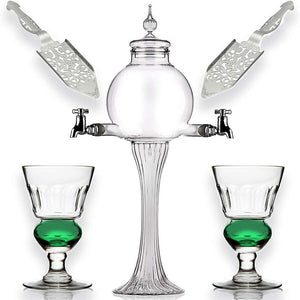This image captures a meticulously arranged, indoor scene set against a pristine white background, creating a stark, floating effect for the objects on display. Centered in the image is an elegant glass dispenser, composed of a tall, tapered base that supports a round, globular bottle. The bottle is topped with a pointed lid, adding a touch of sophistication with its spire-like finial. Two silver faucets extend from either side of the globe, suggesting the dispenser is designed to serve liquids, likely liquor.

Flanking the dispenser are two wine glasses with a unique design: each features a clear glass base and stem, transitioning into a striking green bulb in the middle, and culminates in a trapezoidal bowl for holding beverages. Completing the ensemble, to the upper left and right of the dispenser, sit two ornate, silver cake spatulas. These spatulas are tapered with curved handles and possess a delicate, elevated side profile. Their elaborate, perforated design suggests a decorative yet functional purpose, possibly for guiding the liquid dispensed from the faucets into the glasses below.

This photograph is a study in minimalistic elegance and refined utility, capturing the intricate details of each item against the seamless white background.